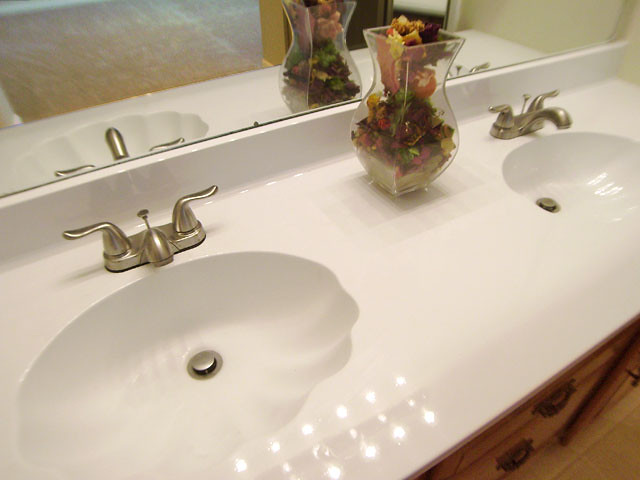This image depicts a modern dual-sink bathroom setup characterized by its clean and symmetrical design. The white countertop elegantly spans the width of the space, providing a sleek surface that complements the twin sinks. Each sink is identical, featuring minimalist fixtures that add to the contemporary aesthetic. Positioned between the sinks is a decorative potpourri vase, adding a touch of natural fragrance and visual interest to the otherwise neutral palette. The overall design is both functional and stylish, encapsulating a sense of simplicity and order.